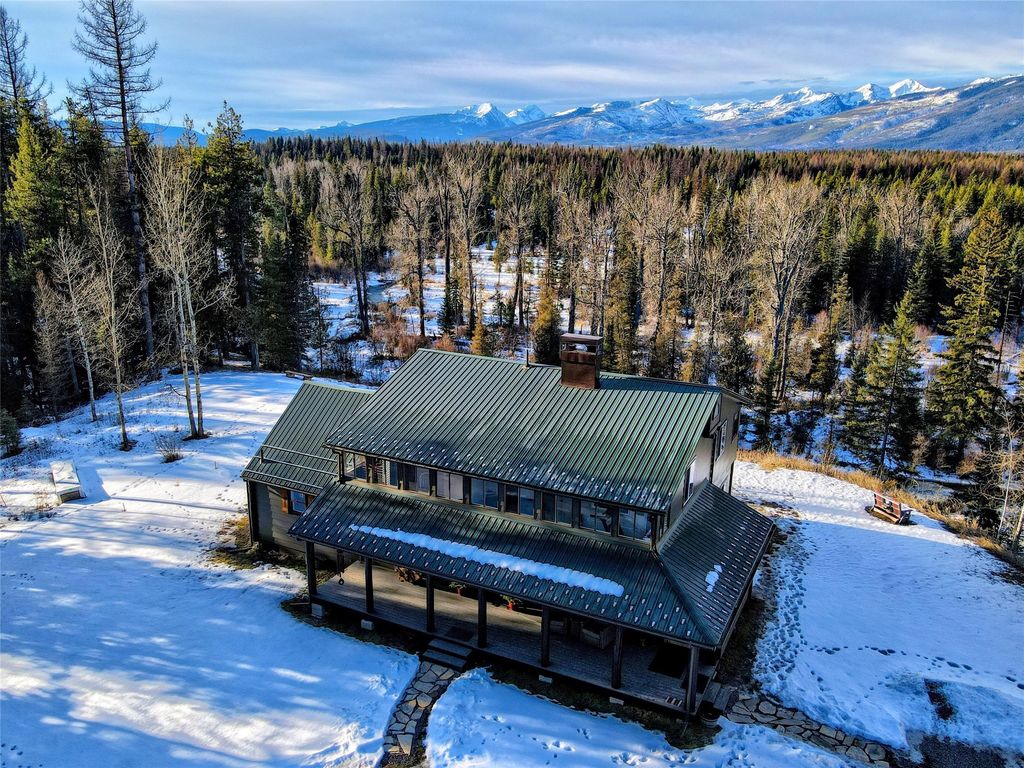A detailed aerial photograph captures a secluded cabin or lodge nestled within a dense forest of green pine trees, framed by majestic mountains in the background. The sky is a blend of light blue and white, suggesting an impending snowfall. The mountains showcase a gradient of colors, with white peaks transitioning into dark blue and gray slopes.

The cabin, situated in a snowy clearing near the bottom of the photograph, exhibits a distinct green roof and a stone path leading from the left side. It's a two-story structure with a brown chimney, two stone walkways, and a wraparound porch. The upper floor has numerous windows, likely indicating bedrooms with scenic views. Closer to the cabin, some trees are bare, emphasizing the winter season. Snow-covered and clear benches provide places to admire the mountainous landscape. Footprints trace paths from the walkway to various points around the house, enhancing the sense of isolation and serenity this lodge offers amid the natural beauty.